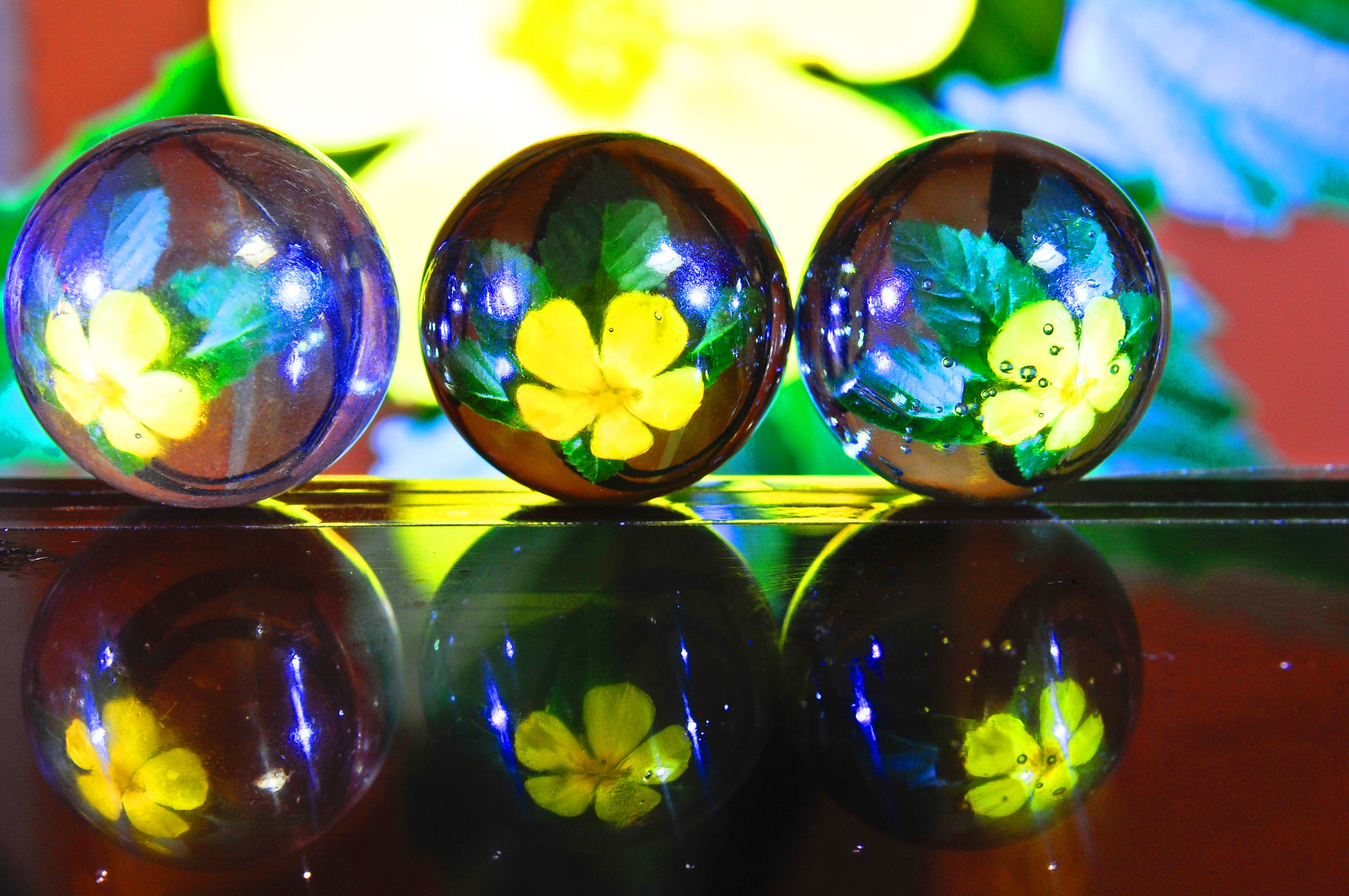This image features three clear, glass-like marbles positioned atop a reflective, possibly glass or laminate surface. Each marble encases a vibrant yellow flower with green leaves, mirroring the flower backdrop which is very slightly out of focus. The yellow flowers inside the marbles, distinguished by their five petals and ornate green leaves, are bright and vivid, with reflections accentuating their luminosity. Light source from the left creates reflections and highlights on both the marbles and the reflective surface they sit on. The backdrop primarily features large painted yellow flowers with darker shades towards their centers, framed by green leaves, set against a predominantly red wall with hints of blue and green accents. The scene appears to be captured indoors with fine details of the marbles and their reflections sharply contrasted by the more subdued, diffused background.